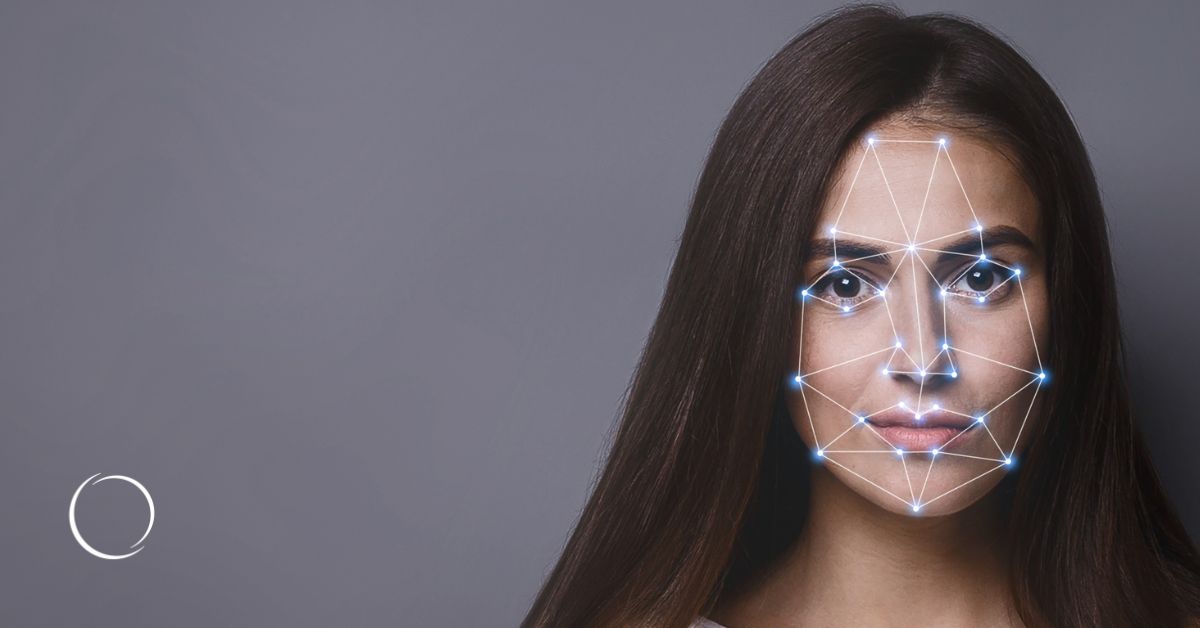The image displays a young Caucasian woman, likely in her mid to late 20s or early 30s, with dark brown hair cascading past her shoulders. The photo is tightly framed, focusing solely on her head and the area just above her shoulders. A series of interconnected blue dots and white lines trace the contours of her face, creating a pattern reminiscent of a facial recognition grid or AI-generated facial map. These geometric lines and nodes highlight her forehead, eyes, nose, mouth, and various facial features, illustrating the mathematical and symmetrical proportions of her face. Her eyes are dark, and she has prominent red lips. The background is a solid steel gray, and a white circle logo is visible at the bottom left, adding a touch of minimalism to the image's aesthetic. The glowing dots give the impression of being illuminated from behind, enhancing the futuristic and analytical feel of the composition.